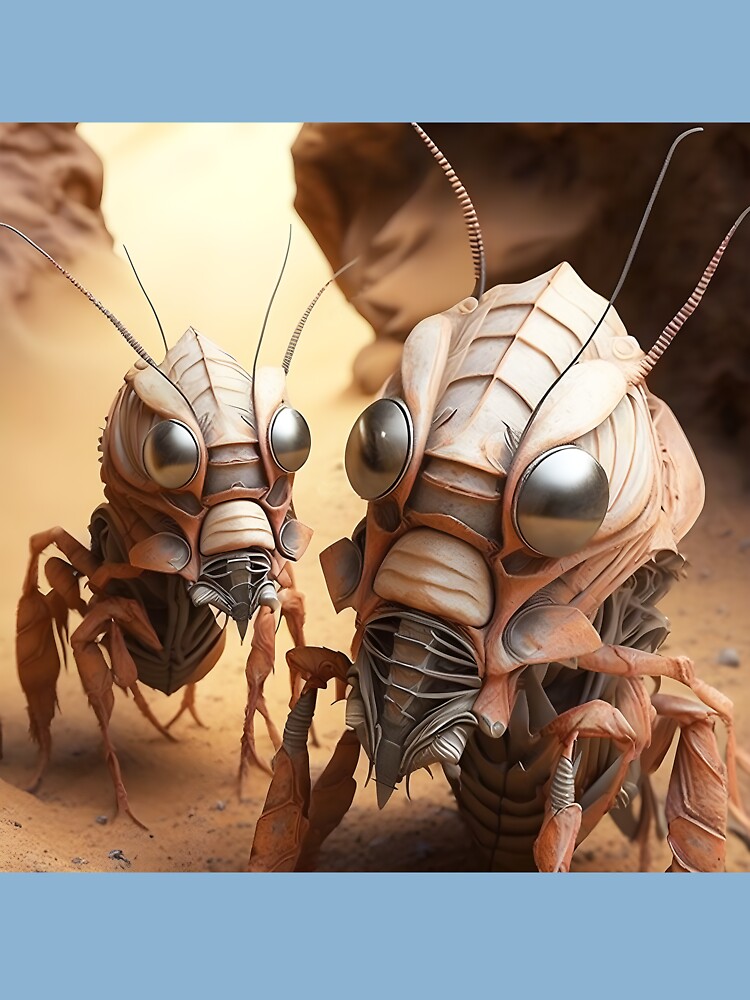The image features a scene with a thick light blue border at the top and bottom, and an animated picture in the center. At the forefront of the scene, there are two large, insect-like robotic creatures set against a desert background replete with brown sand, jagged red clay rock formations, and a sandstorm effect. The creature on the left is turned slightly to the right, while the one on the right faces slightly to the left. Both have mechanical features, including large silver eyes positioned on the sides of their heads, four antennae atop their heads, and what appears to be a metal nose guard characterized by horizontal lines and grill-like protrusions beneath it. Their bodies exhibit a combination of grey and orangish-brown colors, with thick crab-like legs featuring forked toes. The ground underneath them is a dirt pathway interspersed with large stones. The detailed design of these creatures suggests a blend of organic and mechanical elements, enhancing the futuristic, AI-generated feel of the image.